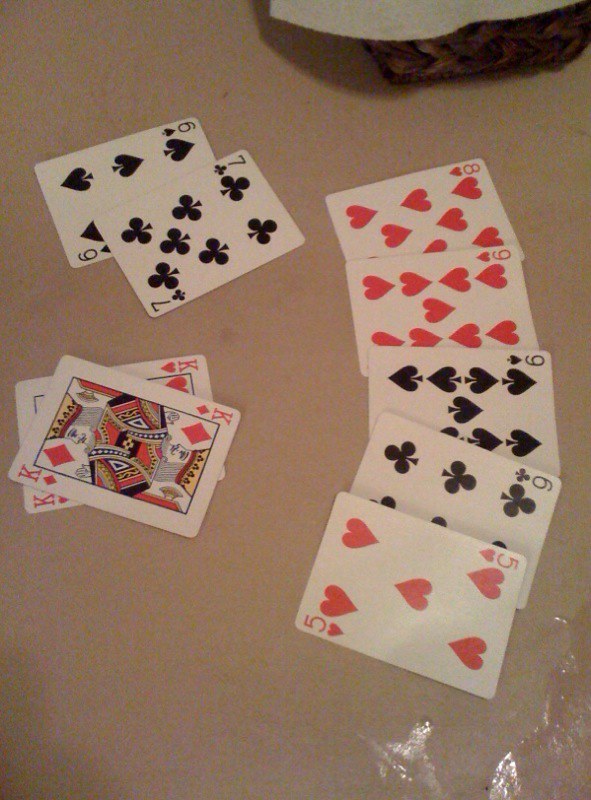The image captures an overhead view of a beige tabletop scattered with an array of playing cards. On the right side, five cards are neatly arranged in a vertical line from the camera's perspective: an eight of hearts, followed by two nines of hearts, a six of clubs, and a five of hearts. To the left of this sequence, two king of diamonds cards are slightly overlaid atop one another, each turned at a slight angle for visual interest. Above the kings, a six of spades partially peeks out from under a seven of clubs, creating a staggered stack. The bottom right corner of the image features a gleaming spot, possibly from a small amount of water on the table. Adding a touch of homeliness, a small brown woven basket sits just above the longest line of cards, holding what appears to be a white washcloth.